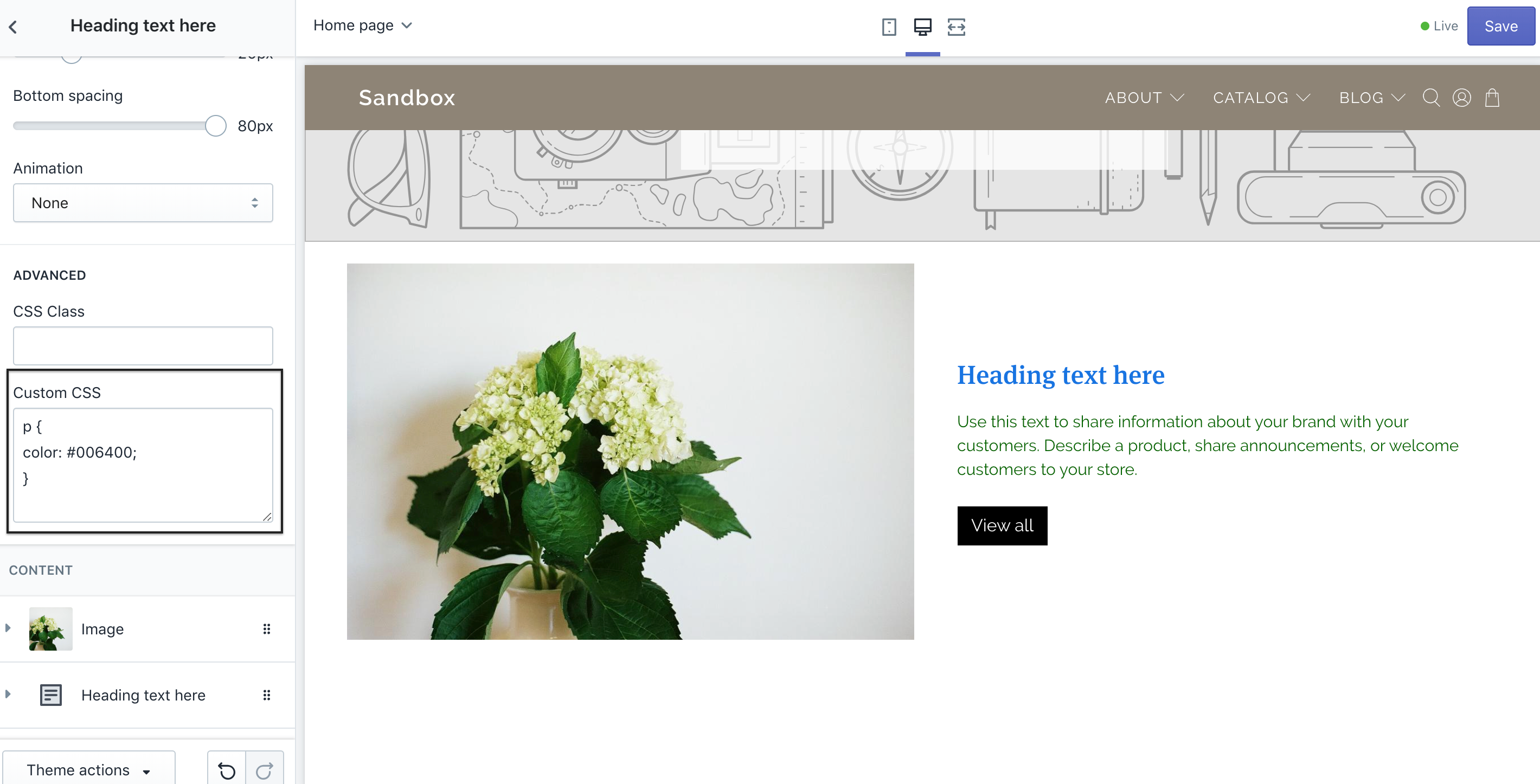This is a screenshot of a website building application called "Sandbox." The main portion of the window features a vibrant photo of a flower arrangement elegantly placed in a vase. Adjacent to this photo is the label "Heading Text Here," accompanied by an empty text input box where a heading can be typed in. On the left-hand side of the screenshot, there is a sidebar displaying multiple customization options available while constructing the webpage. These options include adjusting the amount of bottom spacing, selecting whether to add animations, and a text box for entering various text descriptions. Additionally, there's an image button that allows users to add new images to the webpage, enhancing its visual appeal.